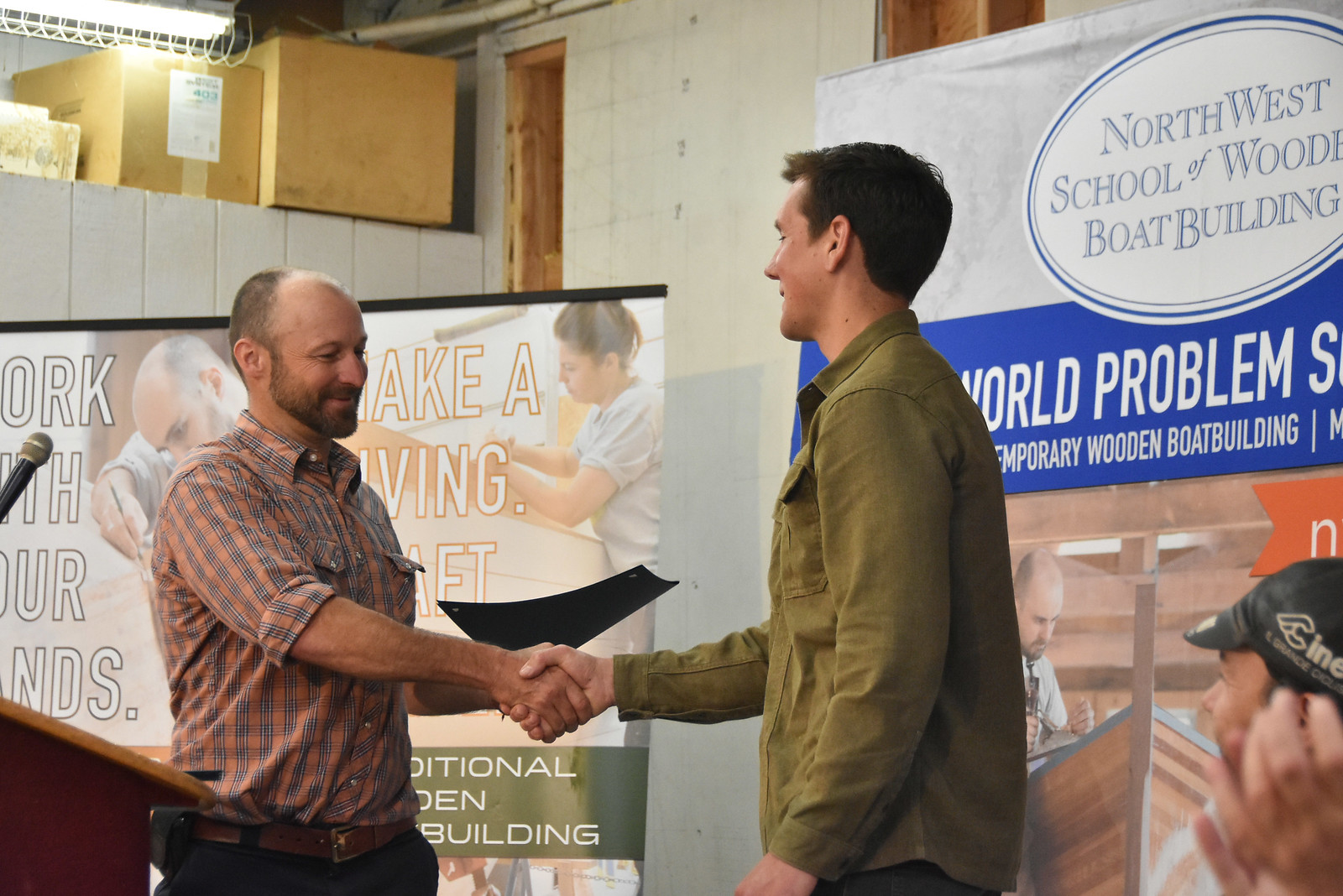In this photograph, captured indoors, likely in a back room or storeroom, two men are shaking hands at the center of the image. The man on the left, standing in front of a podium, wears a rolled-up flannel shirt, revealing his forearms. He has a mostly bald head, with a fringe of hair towards the back, complemented by a mustache and beard. The man on the right, dressed in a dark olive green long-sleeve shirt, has clean-shaven features and dark brown, almost black, hair.

The backdrop includes a series of posters, making the setting appear to be a presentation or awards ceremony. One of the prominent posters, prominently displays the words "Northwest School of Wood and Boat Building" and features an image that appears to depict the man on the left. Additional partial text on the posters reads, "Work with our hands, make a living." The image captures a spectrum of colors including maroon, brown, white, black, gray, green, orange, blue, and white. A couple of other individuals are partially visible in the bottom right corner, further adding to the busy, yet focused atmosphere of the scene.